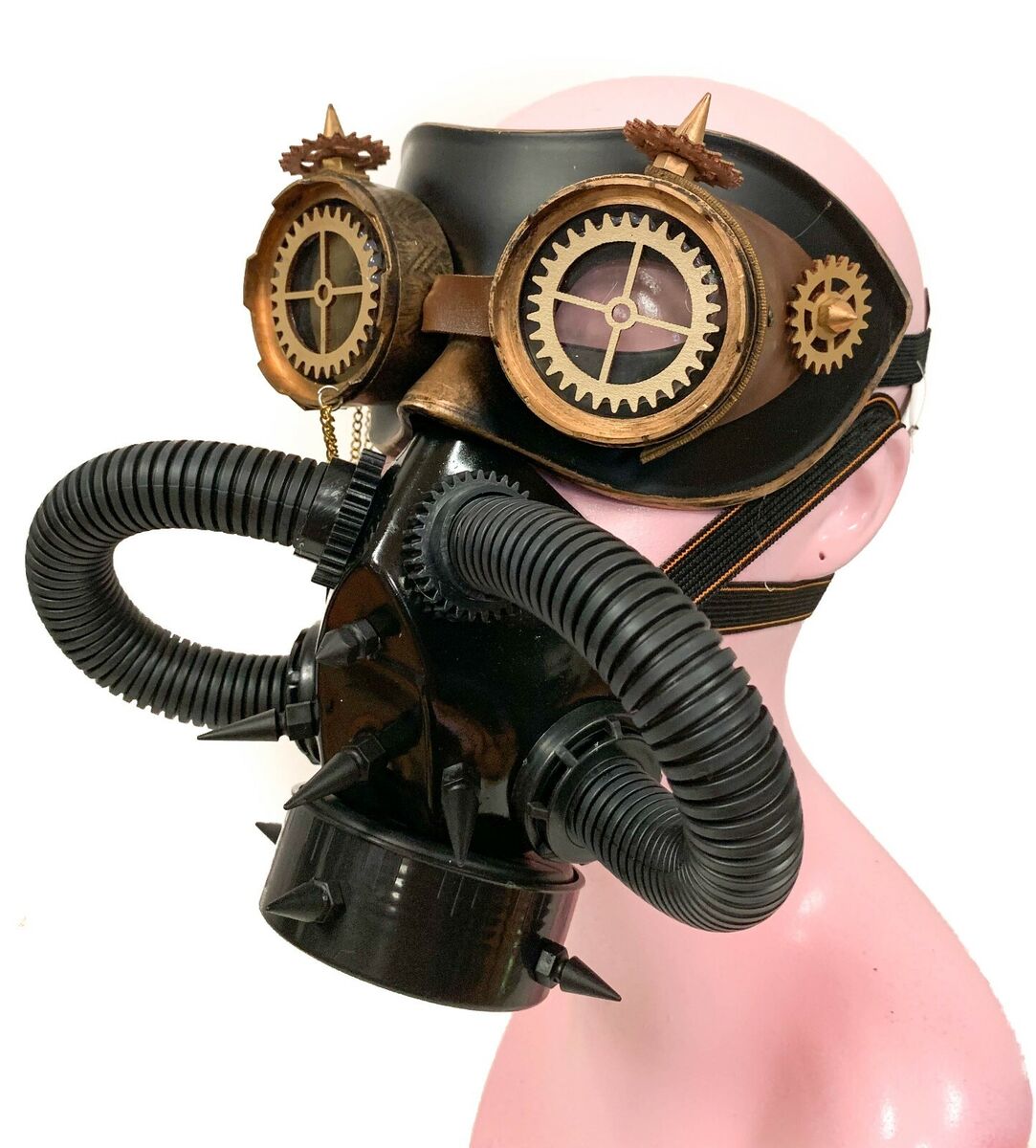The image showcases an intricate piece of artwork displayed on the pink head and left shoulder of a mannequin against a white background. The centerpiece is a heavy-duty, industrial-looking mask that combines elements of a gas mask and a scuba breathing apparatus. The mask features prominent black goggles supported by a bronze-like metal frame with visible gears inside. Above the eyes are two bronze cone-shaped points with gears encircling each one. The nose area is also crafted from a bronze material, giving a cohesive metal appearance around the eye section.

Beneath the eyes, the mask transitions into a black rubber breathing apparatus. Black rubber tubes stretch from beneath the nose to the lower chin area, connecting to a black round canister, likely a breathing filter. The canister is adorned with black spikes, adding to the mask's elaborate and somewhat ominous design. A brown leather strap with gold trim runs around the eyes and the head, and a gold chain with a silver ring connects on the right side of the head. This meticulously detailed and visually compelling mask evokes a sense of antiquity and advanced mechanical design.